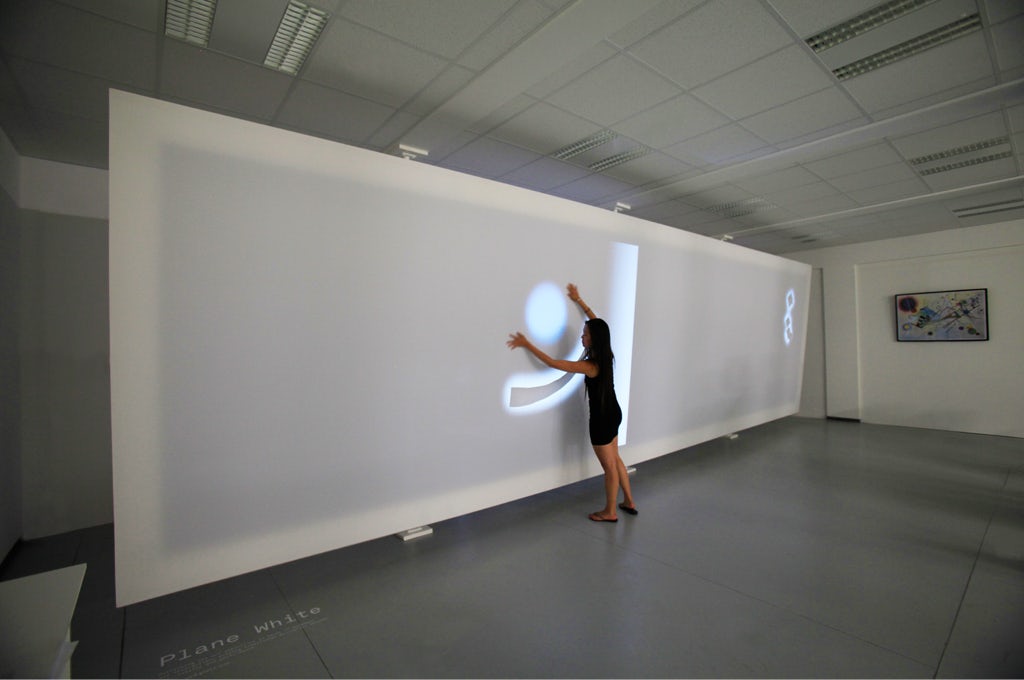The photo captures a vast interior space characterized by its silver tile flooring and grey walls and ceiling. Dominating the entire length of the room is a massive white screen, which appears to be backlit, giving a luminous effect to the area. Standing before this expansive screen is a woman dressed in a sleeveless black dress or skirt. She has her hands raised and positioned against the screen where a round light or glowing sphere is prominently displayed between them. Beneath this circle of light is a horizontal curved bar. To the right side of the screen, there’s an illuminated image of a pillar and lighted chains, and further to the very right of the photo, a painting hangs on the wall. The scene also features some plain white text at the bottom left of the image. The overall ambiance hints at an interactive element, potentially suggesting that the screen reacts to the woman’s hand movements.